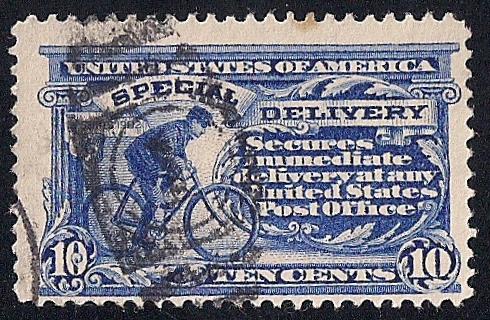This photograph showcases a well-worn, early 20th-century United States postage stamp, predominantly rendered in blue and white hues. Set against a stark black backdrop, the stamp displays its age with visible wear and an ink stain marking its prior use. The centerpiece features a man, dressed in a hat, jacket, and pants, riding a bicycle from left to right. Above the illustration, white letters spell out “United States of America,” while a banner beneath proclaims “Special Delivery.” The phrase “secures immediate delivery at any time United States Post Office” is elegantly nestled within a design resembling vines or plants. The corners of the stamp prominently feature the denomination “10 cents,” each numeral encased within circular, decorative motifs. The stamp's edges are characteristically jagged, indicative of its authentic postal service origin.